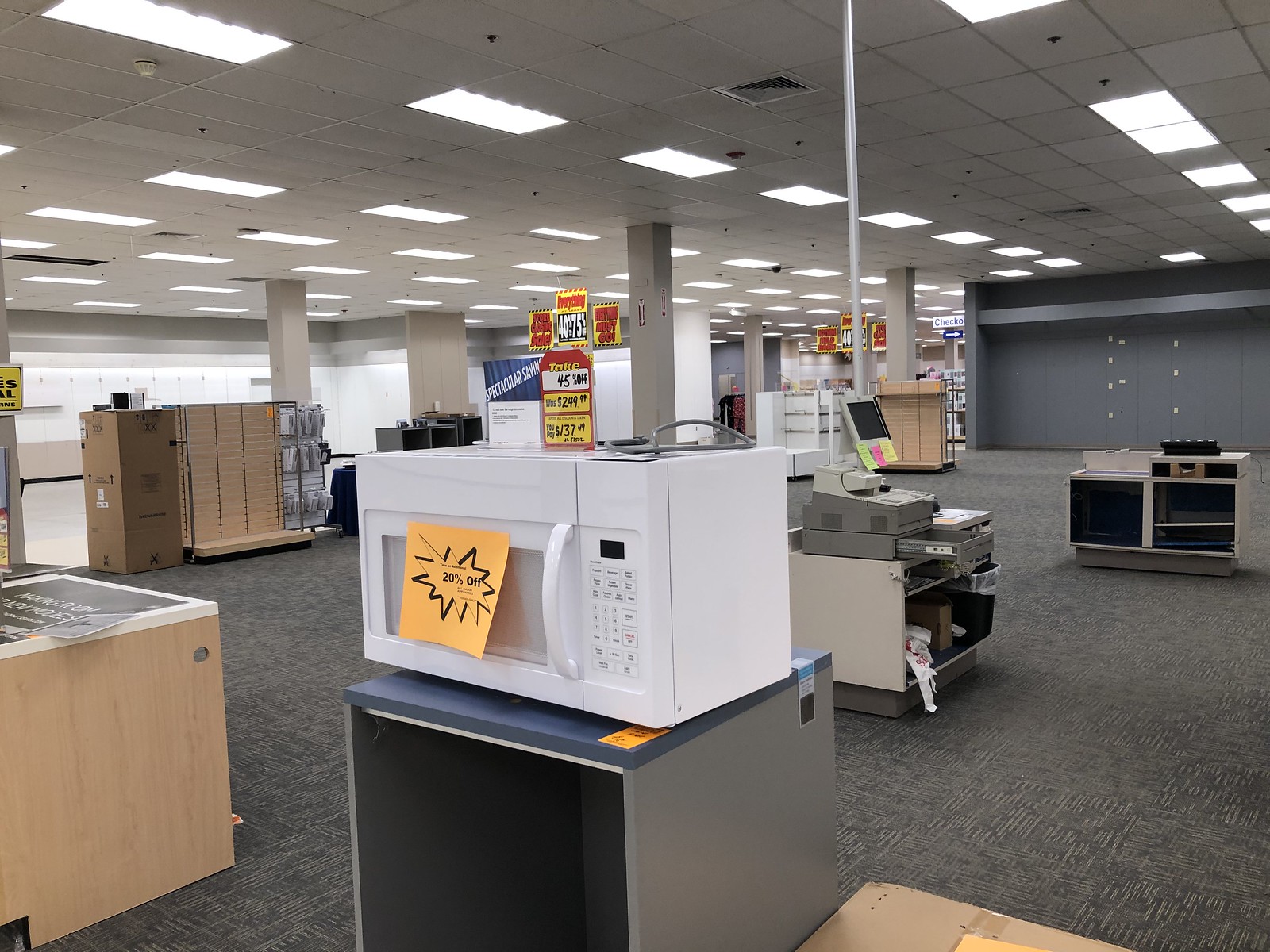The photograph captures the interior of a largely empty department store, depicting a scene suggestive of a liquidation sale. The store, which appears to sell a mix of electronics, furniture, and office supplies, features high ceilings illuminated by numerous fluorescent lights. Central to the image is a white microwave placed on a blue and gray table, adorned with an orange sale sign indicating a 20% discount. Close inspection reveals another label detailing a price reduction from $249.99 to $137.99. Scattered around the microwave are additional varied appliances and a cash register on the right side, marked by a cluster of yellow, pink, and green notes. The surroundings reveal a blend of white linoleum and carpeted floors, with several scattered shelves and a conspicuous large box also visible. Background signs proclaim significant markdowns of 40% to 75% off, reinforcing the notion of an ongoing clearance event. The scene conveys an atmosphere of bustling abandonment, with columns sprouting some separation between remaining stock items in the spacious, fluorescent-lit expanse.